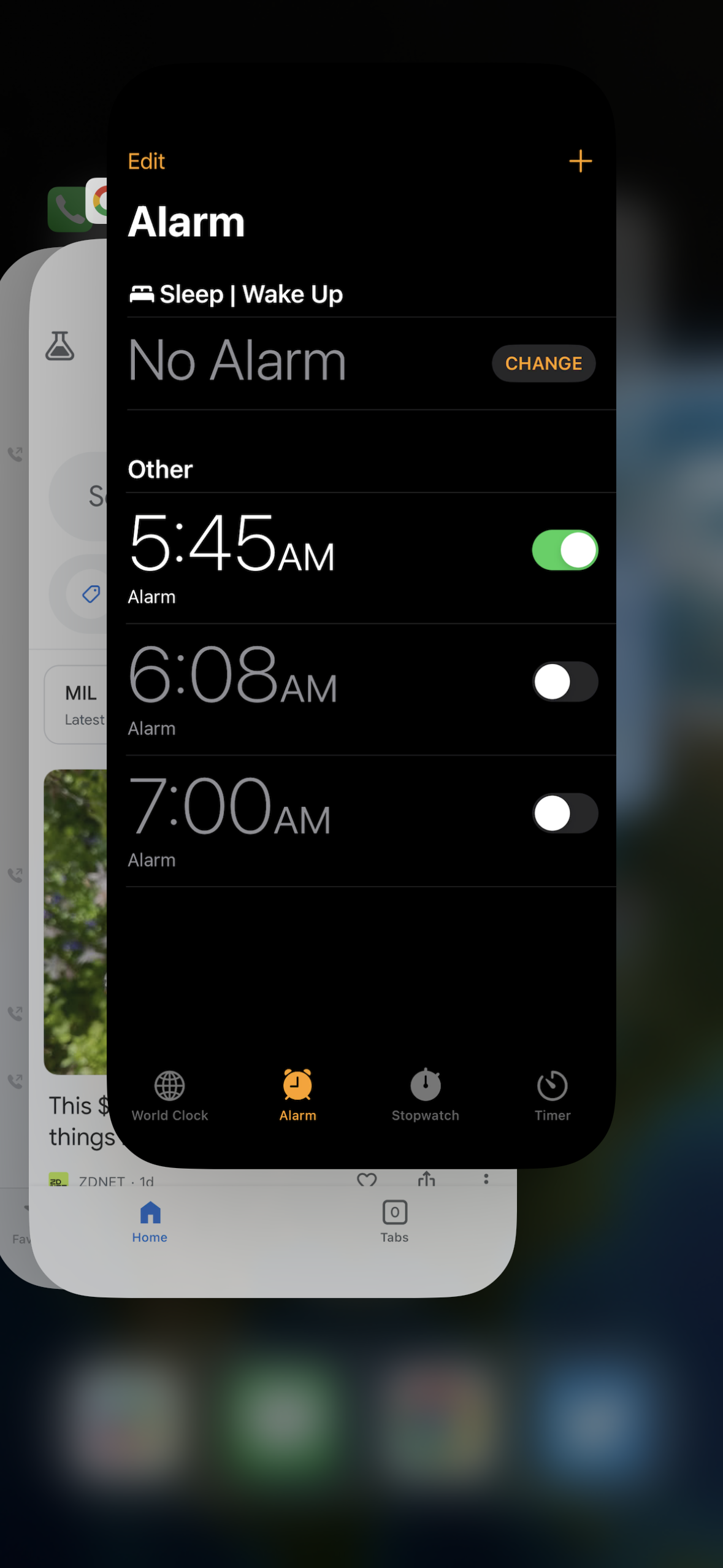The image displays the screen of an iPhone, where the user is in the process of closing all their open apps. The background of the screen is blurred, indicating the multitasking view. Three app windows are visible, layered on top of each other. The foremost app is the Alarm app, showing an active alarm named "Other," set for 5:45 AM and switched on. Additionally, there are two more alarms set for 6:08 AM and 7:00 AM, both of which are turned off. Behind the Alarm app, a partially visible screen hints at a predominantly white interface with a blue home icon at the bottom and an empty tabs indicator, suggesting it might be a web browser with no open tabs. The third app, only slightly visible on the bottom left, shows an outgoing call icon, indicating the phone app is also among those the user is closing.